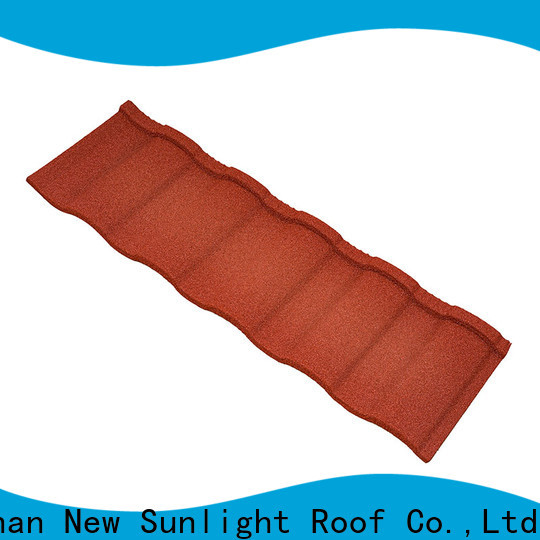The square-shaped image appears to be something you might find on a website. It features a central piece of roof tile against a solid white background, which appears to be an orange-red, terracotta-colored clay roofing tile with a wavy, corrugated pattern. The image may look computer-generated or captured with a slightly fuzzy quality. 

Both the top and the bottom of the image have wavy, blue banners that span across its width. The bottom banner features bold black text, partially cut off, which reads "A.N. New Sunlight Roof CO., LTD." 

The overall composition includes noticeable textures and colors that make the roof tile stand out prominently against the clean, white background. The combination of the wavy blue borders and the bold text adds structure and information about the company, making it clear that the focus is on the distinctive appearance of the clay roof tile.